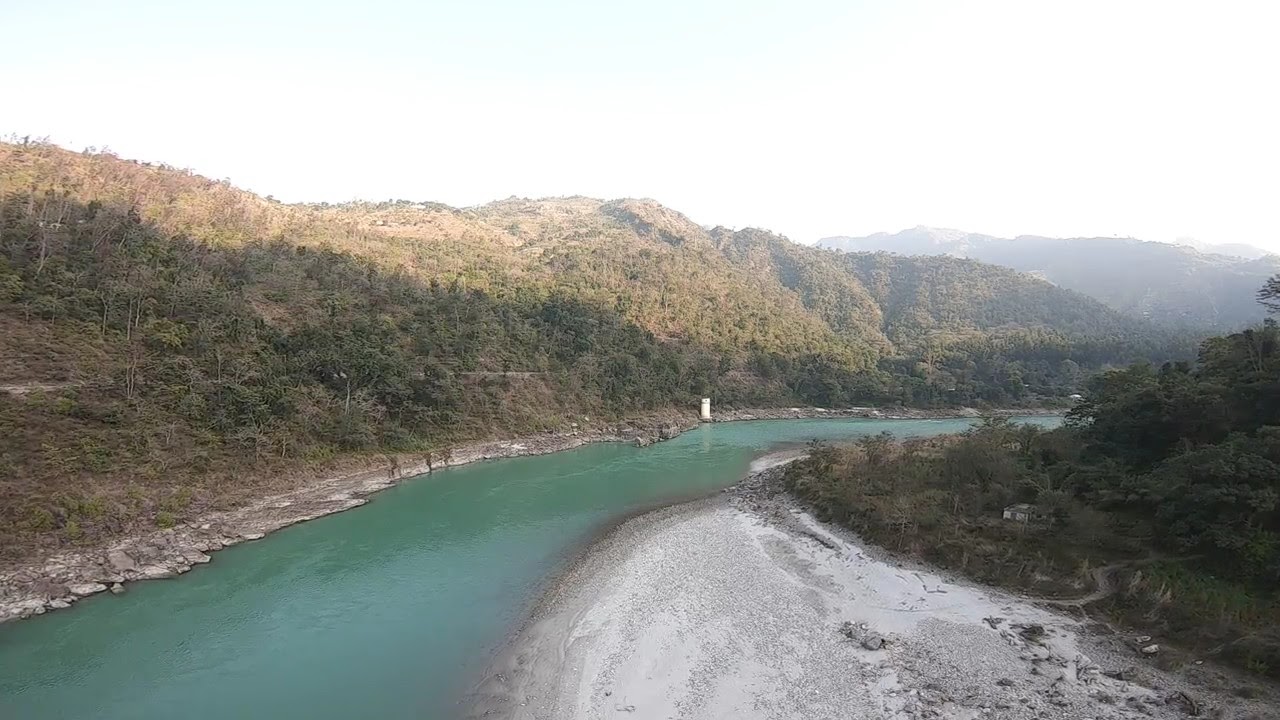In this aerial image, a river with a distinct green-blue hue winds its way through a vast natural landscape, flowing from the lower left corner to the right side. The river is bordered by sandy, gray clay shores and cracked, dirt surfaces. The left bank is home to a white tower, while the lush, green hills on either side are densely covered with trees and green shrubbery. Towards the bottom right of the image sits a small white house with a gray roof, nestled at the foot of a verdant hill. The background showcases additional green, tree-covered hills, all under a sky that transitions from a brilliant blue to a sunlit white. The image captures the serene beauty of this expansive, rugged terrain illuminated by the daylight sun.